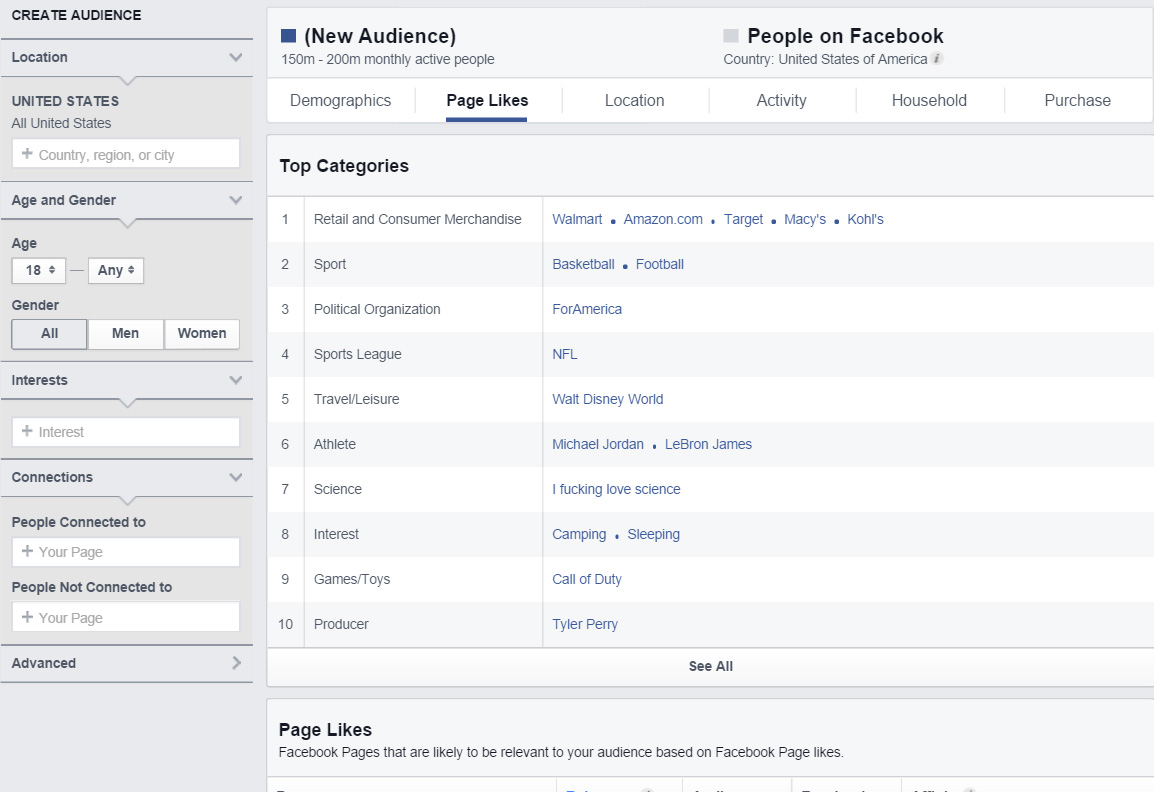The image depicts a detailed interface for creating a target audience. 

On the left side, there's a vertical menu labeled "Create Audience." This menu includes several key sections:

1. **Location**: A drop-down menu is available for selecting geographical areas. Currently, it is set to "United States." Below the drop-down, there is a search bar for specifying locations by country, region, or city.

2. **Age and Gender**: 
   - **Age**: The range is set from 18 to any age.
   - **Gender**: Options for "All," "Men," and "Women" are present, with "All" currently selected.

3. **Interests**: This section features a text input bar for entering specific interests.

4. **Connections**: Here, users can specify connections, with options for "People connected to" and "People not connected to."

5. **Advanced**: An additional section for more granular targeting options.

On the right side, a horizontal menu focuses on "Page Likes." It displays various top categories such as "Retail and Consumer Merchandise," "Sport," "Political Organization," "Sports Leagues," "Travel Leisure," "Athlete," "Science," "Interest," "Games," "Toys," and "Producer."

This descriptive interface allows users to tailor their audience with multiple detailed filters for more effective targeting.